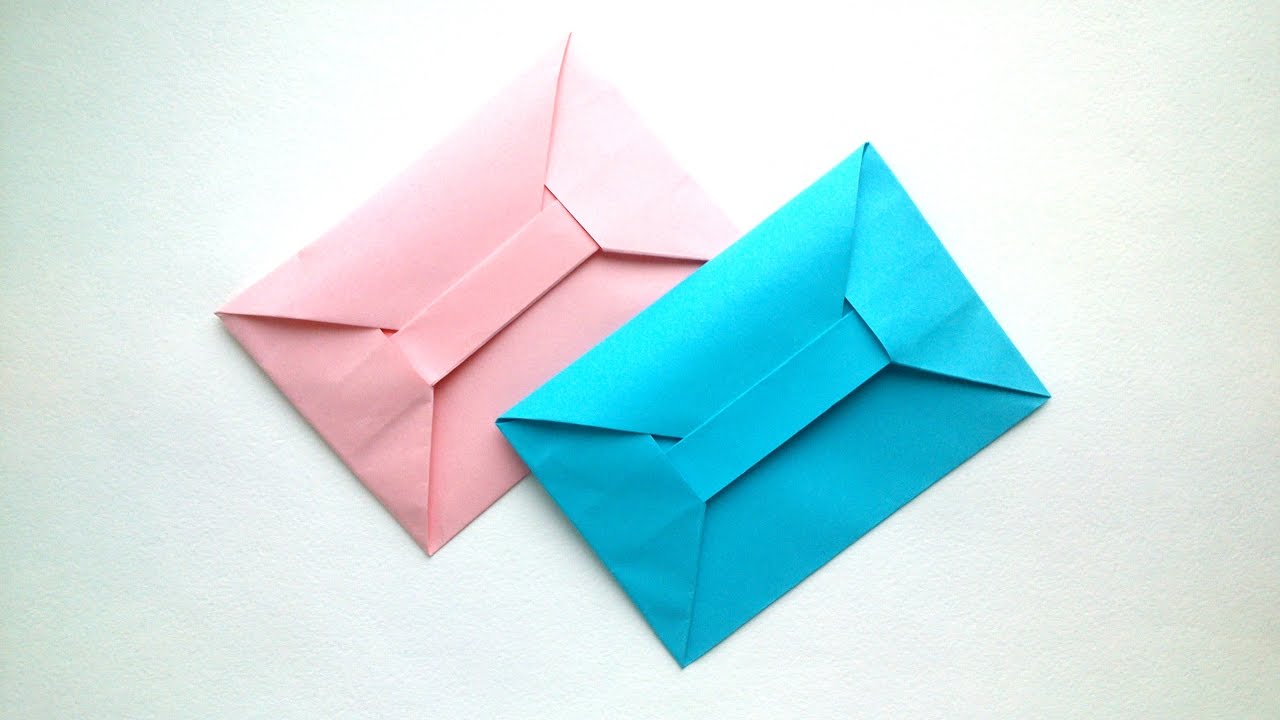This professional overhead photograph showcases two creatively folded envelopes positioned on a pristine white surface. The envelope on the upper left is a light to mid-pink, while the one beneath it is a rich, brilliant turquoise blue. Both envelopes, which could be mistaken for intricately simple origami pieces, feature a unique design: instead of the typical triangle flap, each has an additional horizontal strip of paper crossing the flap, adding to the artistic flair. The pink envelope rests independently, while the turquoise blue envelope's bottom corner slightly overlaps the pink one, creating a harmonious and visually appealing composition. Their unusual folding patterns elevate the mundane envelopes into objects of artistic intrigue.